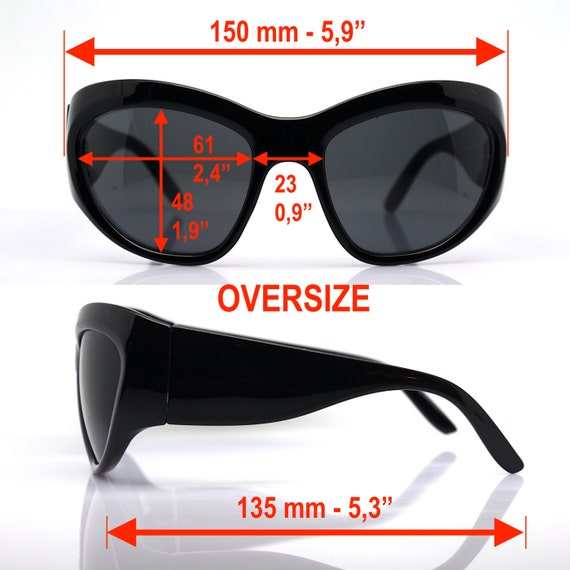This product photograph, designed for commercial listings such as online shops, websites, or catalogs, showcases a pair of stylish black sunglasses with semi-transparent lenses. The background and surface of the image have been edited to appear as a solid white, highlighting the product. The image is split into two halves: the top half presents a front view of the sunglasses, and the bottom half offers a side view.

The front view reveals that the sunglasses feature sleek black plastic frames and lenses with a soft tint. Measurements in red detail the dimensions, with the total width of the frame marked as 150 millimeters (5.9 inches). Additional measurements for the lenses show a width of 61 millimeters (2.4 inches) and a height of 48 millimeters (1.9 inches). The nose bridge width is specified at 23 millimeters (0.9 inches).

The side view provides further insight into the sunglasses' structure, depicting the design from the front of the frame to the back of the ear hook, with the length measuring 135 millimeters (5.3 inches). All numerical details are displayed in bold red, ensuring clarity and visibility against the black glasses and white background. The image is meticulously crafted to emphasize the sunglasses' oversized dimensions and modern aesthetic.